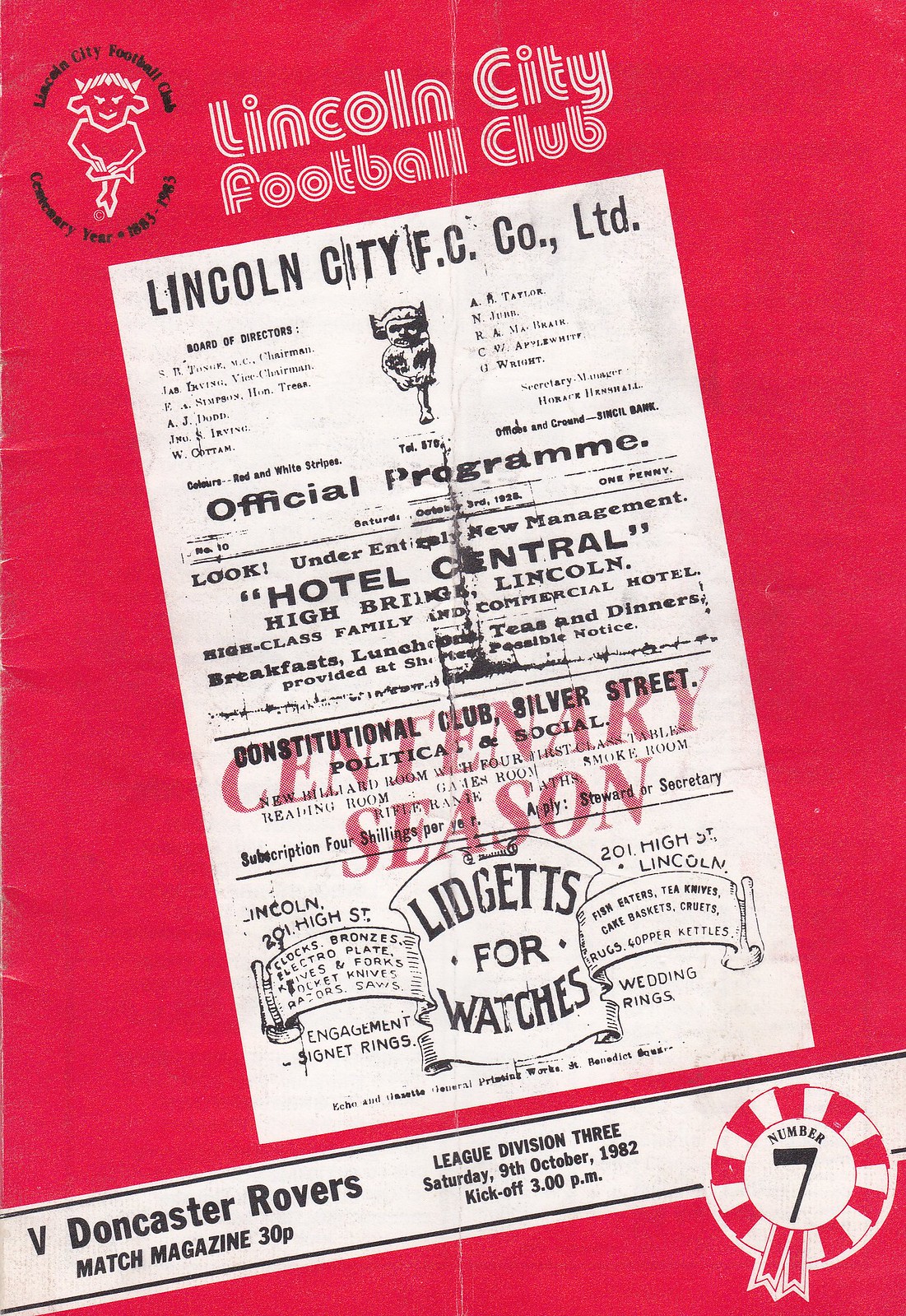This image is a red and white poster for the Lincoln City Football Club, prominently featuring various textual and graphical elements. At the top, "Lincoln City Football Club" is displayed in bold white letters, accompanied by a logo in the upper left corner depicting a white devil or goat-like figure, encased in an oval. Below, the text "Lincoln City FC Co Ltd Official Program" can be seen in a modern print, highlighting the Centenary Season from 1883 to 1983. A white rectangle in the center showcases details such as "Entirely New Management," "Hotel Central," and "Liggetts for Watches" in smaller text. Lower down, the poster indicates an important match: "League Division III, Saturday, 9th October 1982, kickoff 3 p.m." To the left, another white rectangle reads "Doncaster Rovers, Match Magazine, 30p," while in the bottom right corner, a red and white circle sports the number seven. The overall design is pink to reddish-tinted, contributing to the poster's vintage aesthetic.